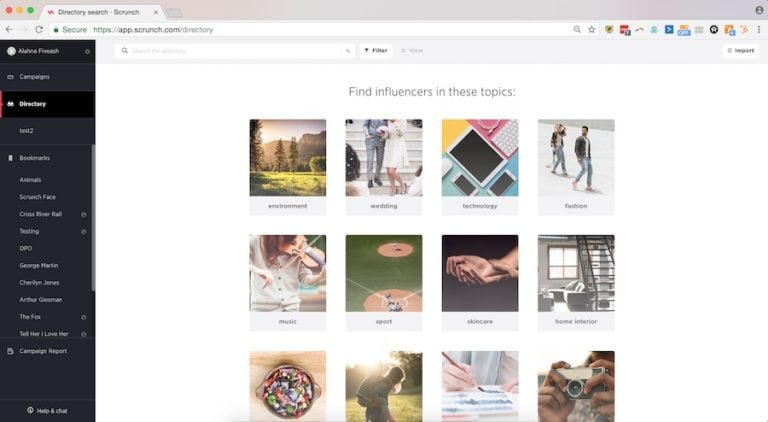This screenshot displays a computer interface for a secure HTTPS app, scrunch.com, focused on directory search. On the left-hand side, there's a black sidebar featuring a list of various items including, "Avila finish campaigns directory, Lent 2, bookmarks, animals, scrunch face, cross river road, testing, QPO, George Martin, Cheryl Jones, Arthur Graham, the fox, tell her I love her, and campaign report."

The main section of the screen showcases 12 pictures, each representing different categories for finding influencers. These categories and their corresponding images are:

1. **Environment**: A scenic view of a mountain range with trees and a grassy meadow.
2. **Weddings**: The lower part of a bride and groom descending church steps together.
3. **Technology**: An assortment of tech devices including two smartphones, a computer keyboard, and a tablet.
4. **Fashion**: Two people dressed in blue jeans and white t-shirts with flannel shirts over them.
5. **Music**: A man in a white sweater playing the violin.
6. **Sports**: A baseball diamond.
7. **Skin Care**: Cupped hands, suggesting care and treatment.
8. **Home Interior**: A set of open stairs with a visible living room in the background.
9. **Food**: An image cut off but identifiable as a bowl of candy.
10. **Artistry**: A girl painting.
11. **Photography**: A guy holding a camera.
12. **Travel/Adventure**: A girl wearing a backpack, presumably indicating travel or exploration.

Each of these images helps to identify the relevant influencers for the depicted topics.